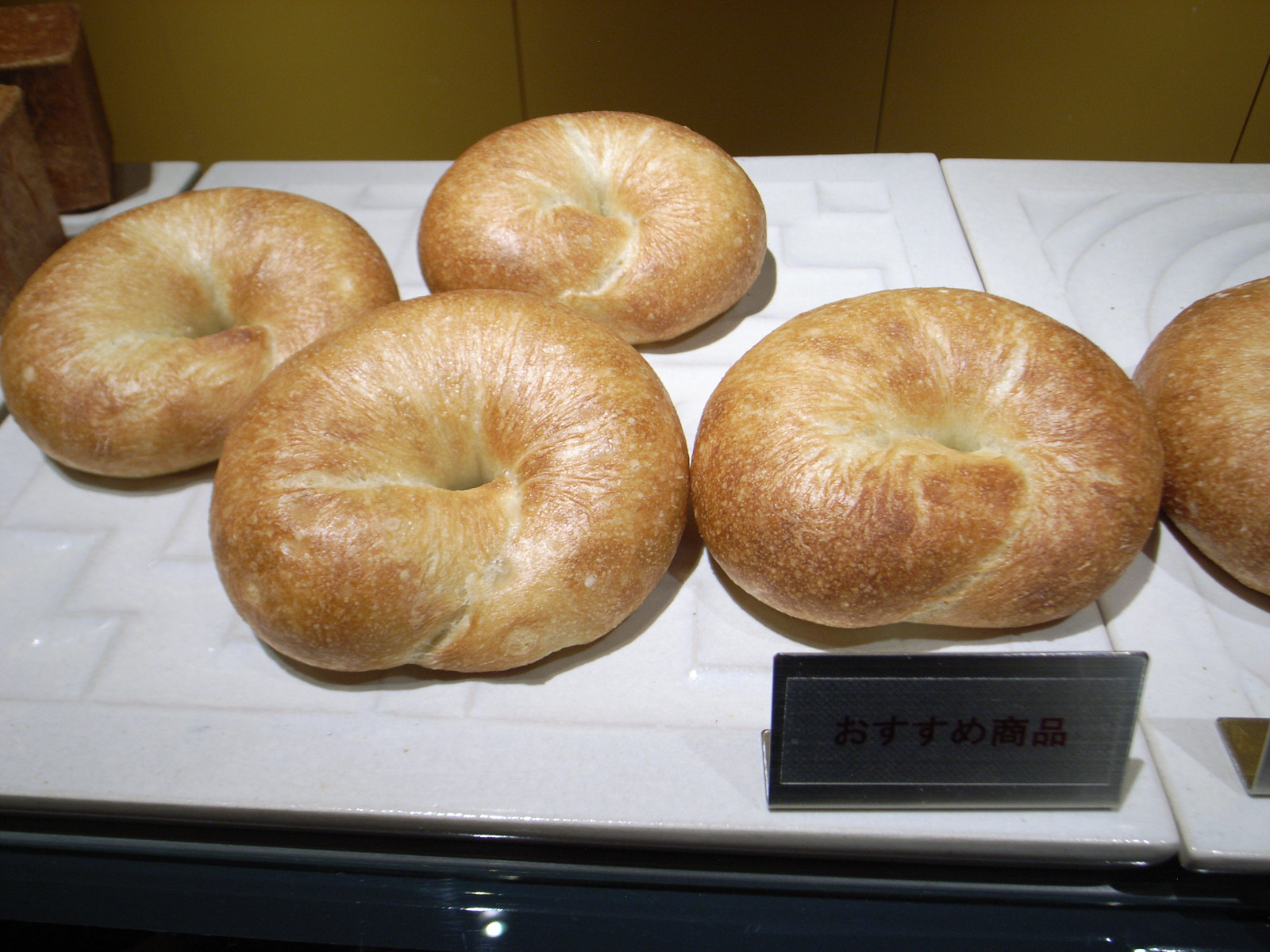The image showcases a bakery display area, possibly located in the Far East, featuring a horizontal rectangular photograph with a distinctively warm and inviting aesthetic. At the forefront, five uniquely-shaped, golden-brown rolls are placed on a sleek white surface, arranged in a visually appealing semi-circle. These rolls resemble puffed-up croissants or bagels with a textured, ring-like appearance and indented centers, resembling belly buttons. Each roll has a glossy brown glaze, suggesting a crispy exterior that would pair well with butter and cheese.

The white rectangular plates with geometric designs holding the rolls rest on a black countertop or table, providing a stark contrast that highlights the baked goods. A small stainless steel plaque with black Asian characters, likely either in hiragana or kanji, is positioned at the bottom right, hinting at their exotic origin. In the background, a golden-brown wall with indistinct brown squares can be seen, adding to the cozy ambience of the bakery. The entire setup appears meticulously curated to entice customers with its fresh and delicious display.